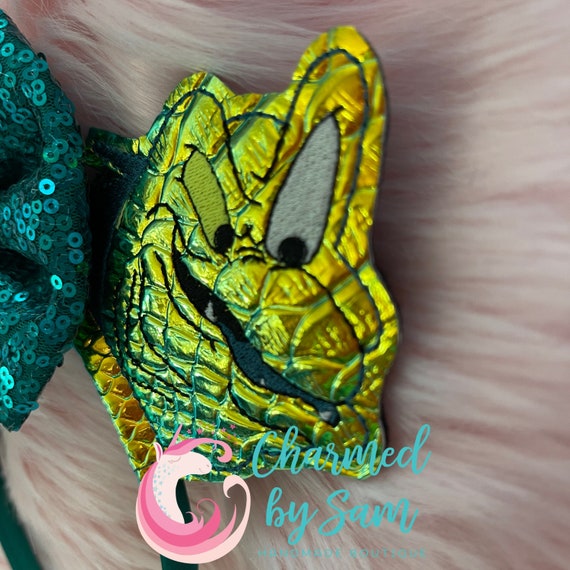This image is a promotional advertisement for an arts and crafts vendor named "Charmed by Sam." The photo showcases a close-up of a headband adorned with a character that resembles the Grinch from Dr. Seuss. The character's face is crafted from shiny, metallic, or gold fabric and features distinctive details such as yellowish-gold scales, large black-stitched mouth, and mismatched eyes—one yellow and one white with black pupils. At the bottom of the image, there is a logo depicting a pink unicorn with a mane composed of varying shades of pink, accompanied by the blue text "Charmed by Sam." The background is adorned with a combination of elements, including green sequin fabric and a fur pillow with sweeping pink and white strokes, adding to the whimsical and eye-catching visual appeal of the advertisement.